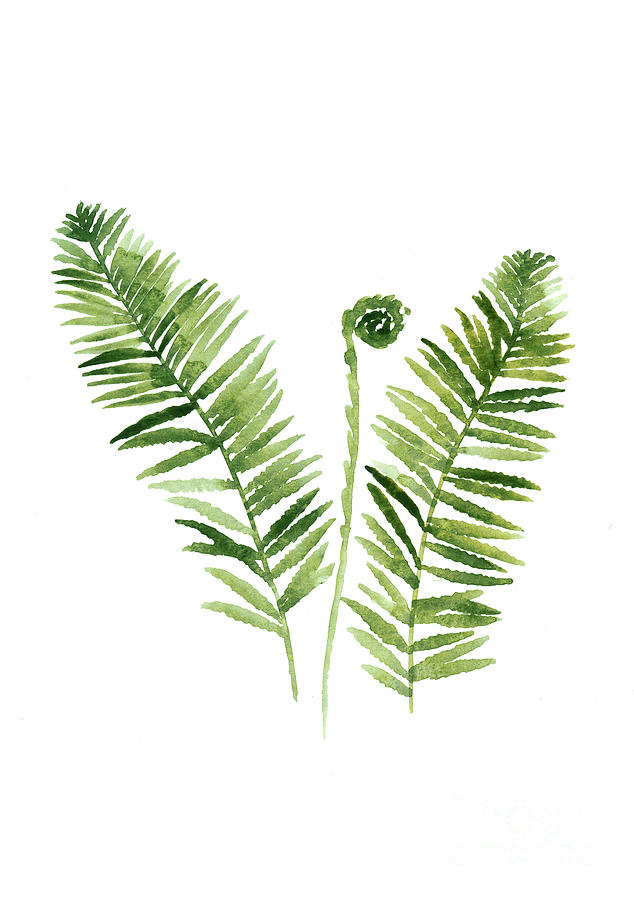This is a high-quality watercolor illustration of a typical fern showcased on a white background. The artwork features three distinct fern fronds: two mature leaves positioned on the left and right, and a smaller, immature frond situated in the middle, characterized by a long, skinny stem curled at the top without foliage. The mature leaves are composed of numerous individual leaflets branching off from the central stem, creating full foliage. The colors are rendered with great accuracy, presenting a range of green hues, from lighter greens at the base to darker evergreen pops throughout. The overall execution of the piece demonstrates exceptional skill in watercolor technique, with precise lines and vibrant, harmonious color tones.